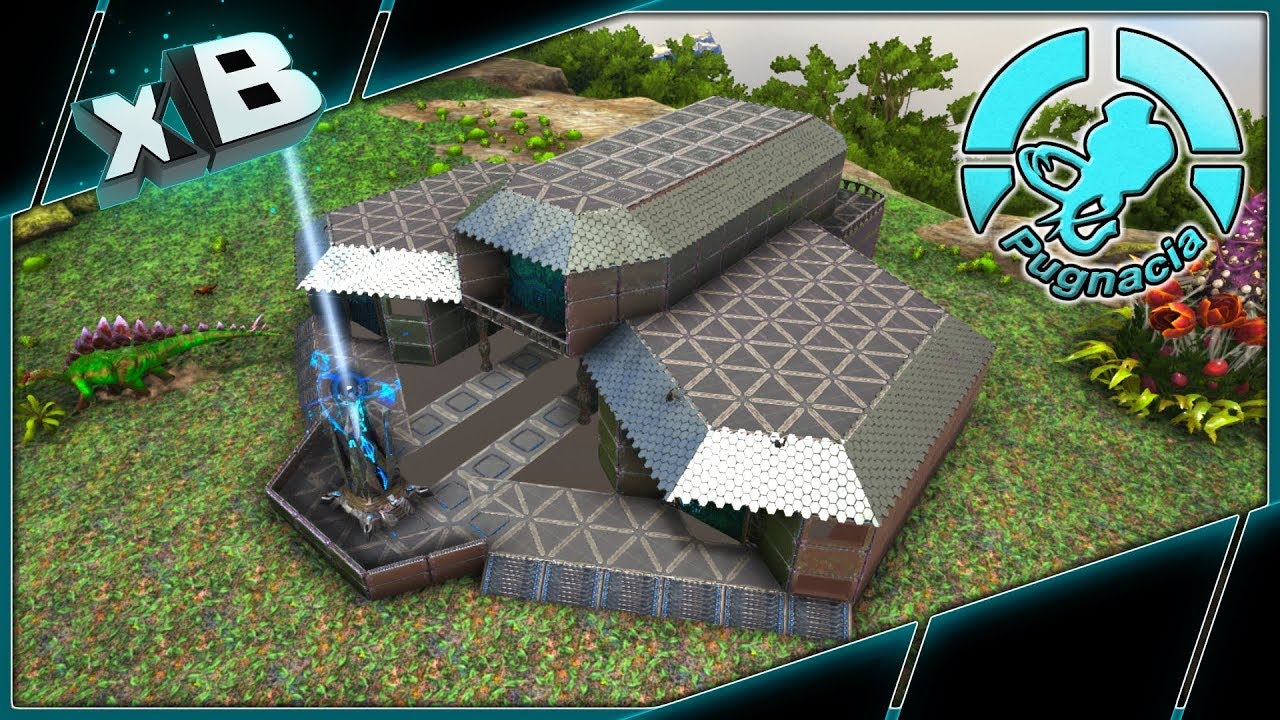The image titled "Pugnacia" features a highly detailed and geometric 3D model, possibly from a video game or digital art project. The scene is set on a grassy plateau accented with flowers in the right corner. Positioned prominently in the center is a steel gray, futuristic building, split into three segments, giving it a sophisticated, modern appearance. To the front of this building, a beam of light descends from the white letters "XB" in the top left corner, targeting a blue-hued, transformer-like creature. This creature, composed of varying shades of blue, appears to be either teleporting in or out of a pad. Adjacent to this creature on its right is a dinosaur, resembling a brontosaurus, vividly colored in green and red. The top right corner of the image features a logo that reads "Pugnacia" in a teal color, accompanied by the silhouette of a woolly mammoth or elephant head with large tusks, adding a touch of intrigue and fantasy to the scene.